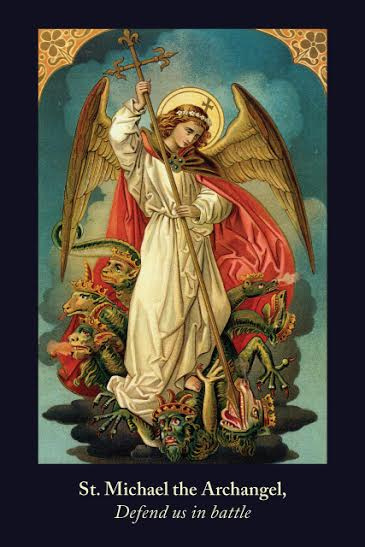This image, labeled at the bottom in italic white letters with "Saint Michael the Archangel, defend us in battle," portrays a dramatic painting of St. Michael. He is depicted wielding a large staff or scepter, topped with what appears to be three fleurs-de-lis, using both hands to spear a demon-like creature with a lizard or dragon head adorned with a crown. The saint, standing on a multitude of similar dragon-like creatures, exudes authority and power. One creature writhes in pain under his foot while another, positioned behind him, emits steam. Additional dragon heads are visible, emerging from both the left and right sides of the artwork. St. Michael is adorned in a white gown, a red flowing cape, and a headband with a cross. His large cream-colored wings extend from his back, and a yellow halo graces his head. The backdrop of the image is black, emphasizing the vivid and dynamic scene, further framed by the black borders that encapsulate the artwork.